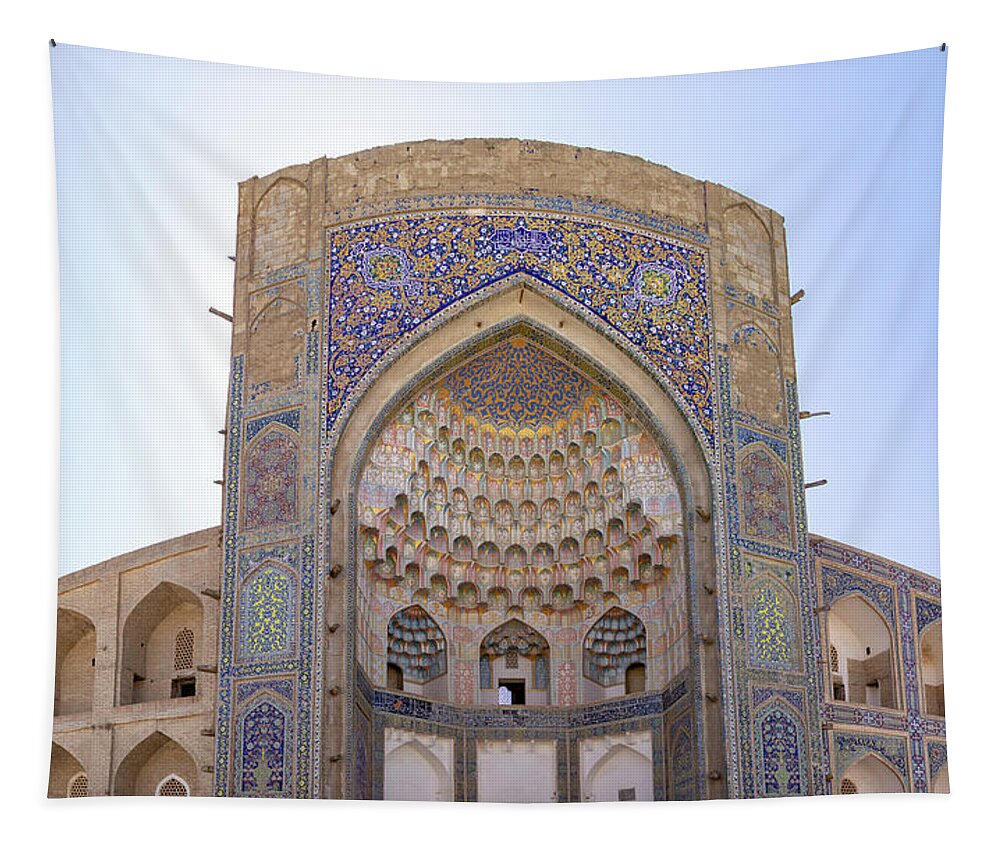The image depicts a beautifully intricate tapestry, hung with black pins in the upper corners, which appears to portray a large, ornate building reminiscent of Middle Eastern Muslim architecture. The building, adorned with detailed patterns of royal blue, yellow, and orange tiles, features multiple stories, with a prominent central section flanked by smaller rectangular areas filled with tiles. The structure showcases numerous arches, some with triangular tops, and windows or balconies that add to its elaborate design. The backdrop includes a vividly painted blue sky with scattered clouds, enhancing the overall elegance of the tapestry. Wrinkles in the fabric suggest it could be made out of cloth or a similar material, possibly sold as a blanket, poster, or banner. The architecture bears a striking resemblance to a mosque or a temple, highlighting its meticulously crafted beauty.